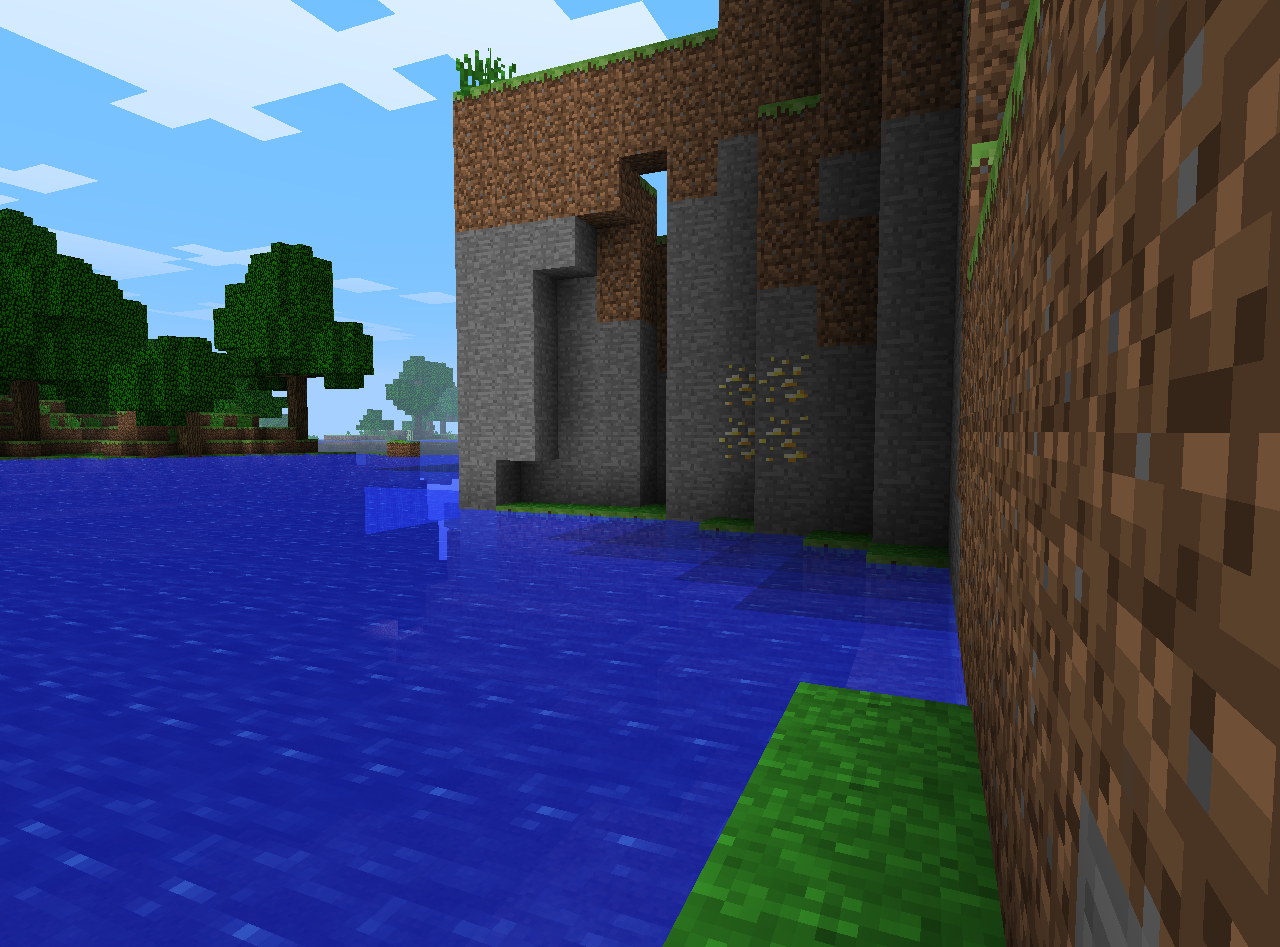In a visually striking scene from a block-based video game reminiscent of Minecraft, the image captures a serene natural landscape. Dominating the foreground is a vast expanse of blue water, perfectly mirroring the cloudy sky above. To the left, a small, densely forested island boasts lush green trees, offering a stark contrast to the water's blue. On the right, a towering cliff made of earthy brown soil and rugged gray stone dramatically extends into the water. Portions of this cliff have been intricately cut away, unveiling a complex network of internal structures. These exposed layers reveal an assortment of materials, including valuable ore deposits ripe for mining. A prominent entrance at the cliff face suggests the possibility of a cave or mine waiting to be explored. The entire scene is rendered in the game's signature pixelated textures, adding to its nostalgic charm.